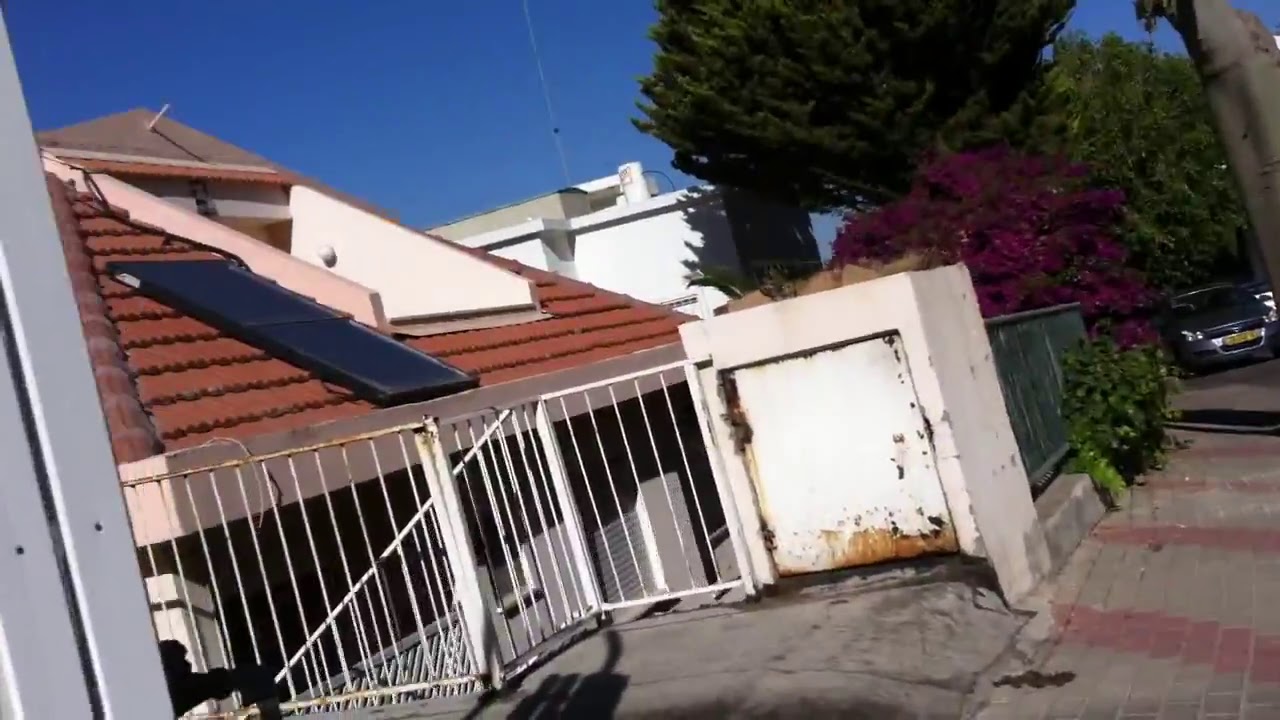The photo captures the exterior of a residential property, taken from an angled perspective that gives the scene a tilted appearance. On the right side of the image, a stone pathway leads up to a dark-colored car parked at its end. Surrounding the car are various trees and bushes, adding greenery to the scene. The property is encased by fencing, which includes a white concrete structure with a small, rusted door resembling a dog kennel.

Beyond this fencing, the land slopes down to reveal a house with a pottery-colored roof, featuring an embedded balcony and a large solar panel connected via a cable. The house, somewhat obscured by darkness, displays windows and a doorway beneath the solar panel. To the far right, a public footpath made of paving blocks with red diagonal lines runs alongside the scene, extending towards the distant silver car with a yellow license plate. The image is rich with natural elements, including various trees and bushes that frame the house and its surroundings.